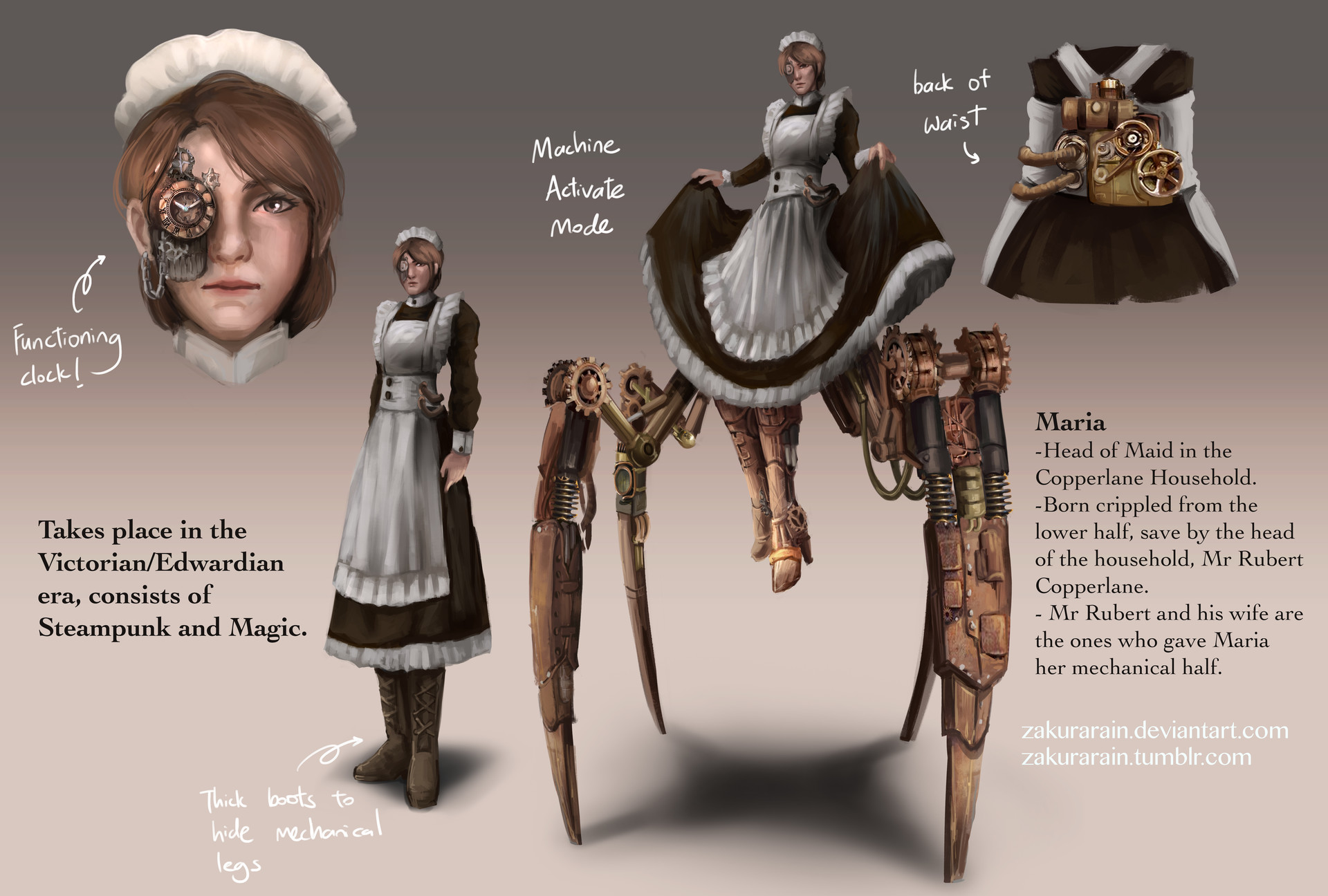This digitally generated image, likely created for educational or narrative purposes, depicts a white woman with short brown hair adorned in a vintage maid or nurse outfit reminiscent of the Victorian and Edwardian eras. A notable feature is her detailed headgear, which includes a functioning clock embedded in one eye and fixed through her ear. In her attire, a knife is conspicuously inserted into her gown, which she lifts to display her boots and mechanical limbs. The caption explains that she is Maria, the head maid of the Copperling household. Born with a crippled lower half, Maria was saved and augmented with mechanical limbs by Mr. Robert Copperling and his wife. These mechanical limbs include four spider-like appendages equipped with sharp ends, shock absorbers, and rotators, activated in "machine mode." The image includes various descriptive elements such as "functioning clock," "Victorian and Edwardian era," "steampunk and magic," and "thick boots to hide mechanical legs." Additional close-ups highlight the controls on her waist belt. The source of the image is credited to ZekirianDeviantArt.com and ZekirianTumbler.com.